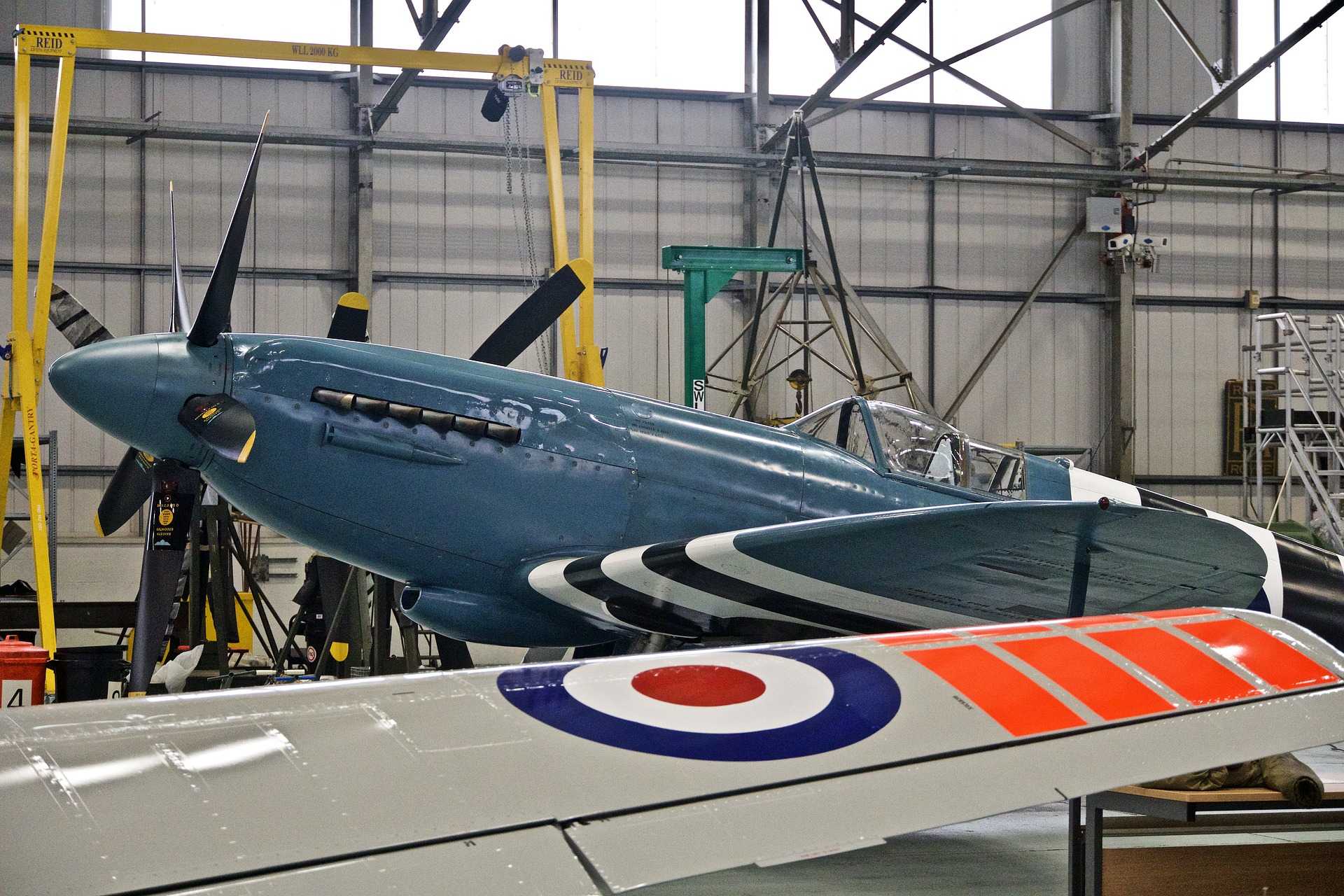In this detailed photo taken inside a metal aircraft hangar, a vintage blue airplane with a front propeller is prominently featured. The plane’s wings are marked with distinctive black and white stripes. In the foreground, partially obscuring the blue plane, is the wing of another aircraft. This gray wing is adorned with a colorful bullseye pattern – blue, white, and red in the center – as well as several orange stripes. The surrounding hangar is noticeably bright due to daylight streaming through windows positioned high around the perimeter. The background reveals various pieces of equipment, including metal ladders and beams. Additionally, there’s a hint of a yellow object with vertical beams, possibly serving as anchor supports, adding to the intricate details of the busy hangar environment.